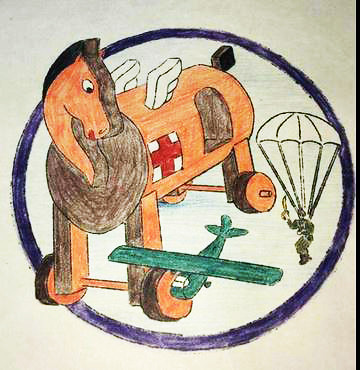The image is a detailed, hand-drawn depiction on white paper, apparently created with colored pencils or crayons, resembling a child's artwork. The central focus is a toy-like hobby horse made of wood with rounded features. The horse, colored in a reddish-brown hue with darker brown shading, stands on wheels connected by small dowels and has white wings attached to its back. Its head, adorned with a short black mane, is turned to the right, revealing a small diamond-shaped dark brown tail at the rear. A distinctive white square with a red cross marks its side, suggesting a medical theme.

Encompassing the horse is a bold black circle with a blue-purple fill, which dominates the composition. Within this circle, the horse is surrounded by other elements: Positioned to the left, a vintage green airplane with a white cockpit extends its wing straight across. Above and slightly to the right of the airplane, a soldier in dark green, equipped with a white parachute, appears in the midst of parachuting down, holding what seems to be a knife or weapon.

Every component of the drawing contributes to the theme of playful imagination, while the intricate details and vibrant colors bring the scene to life.